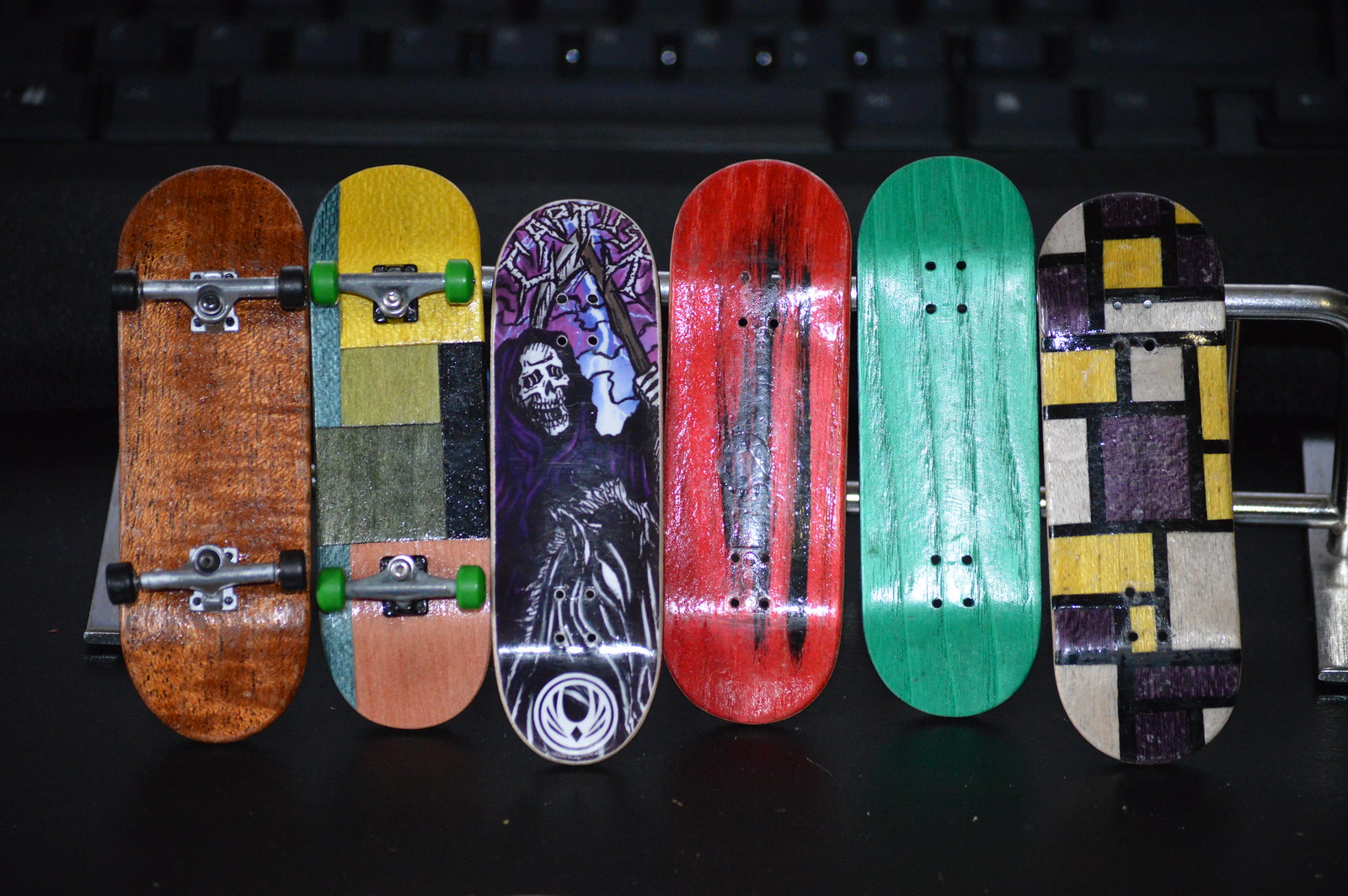This colour photograph features six miniature skateboards, likely of the Tac-Dac brand, positioned side-by-side against a silver, chrome display stand. The background displays a black computer keyboard, suggesting the skateboards' small size. Detailed descriptions of the skateboards from left to right are as follows:

1. The first skateboard has a medium brown wood finish with no additional design, featuring black wheels and gray gear.
2. The second skateboard showcases a multicolored patchwork design with distinct sections of yellow, green, gray, black, peach, and blue. It has green wheels and gray gear.
3. The third skateboard has a vivid purple background with an image of the Grim Reaper wielding a scythe, complemented by lightning elements.
4. The fourth skateboard is red with black smears and occasional white streaks, giving a dynamic appearance.
5. The fifth skateboard is turquoise with a wood grain texture, presenting a blue-green hue.
6. The final skateboard has a checkered pattern with squares and rectangles in purple, yellow, white, and black outlines.

Two of the skateboards, specifically the ones on the left, are positioned upside down, showing their wheels, while the rest face upwards. The background beyond the display is dark, with hints of small round objects visible near the top of the image.